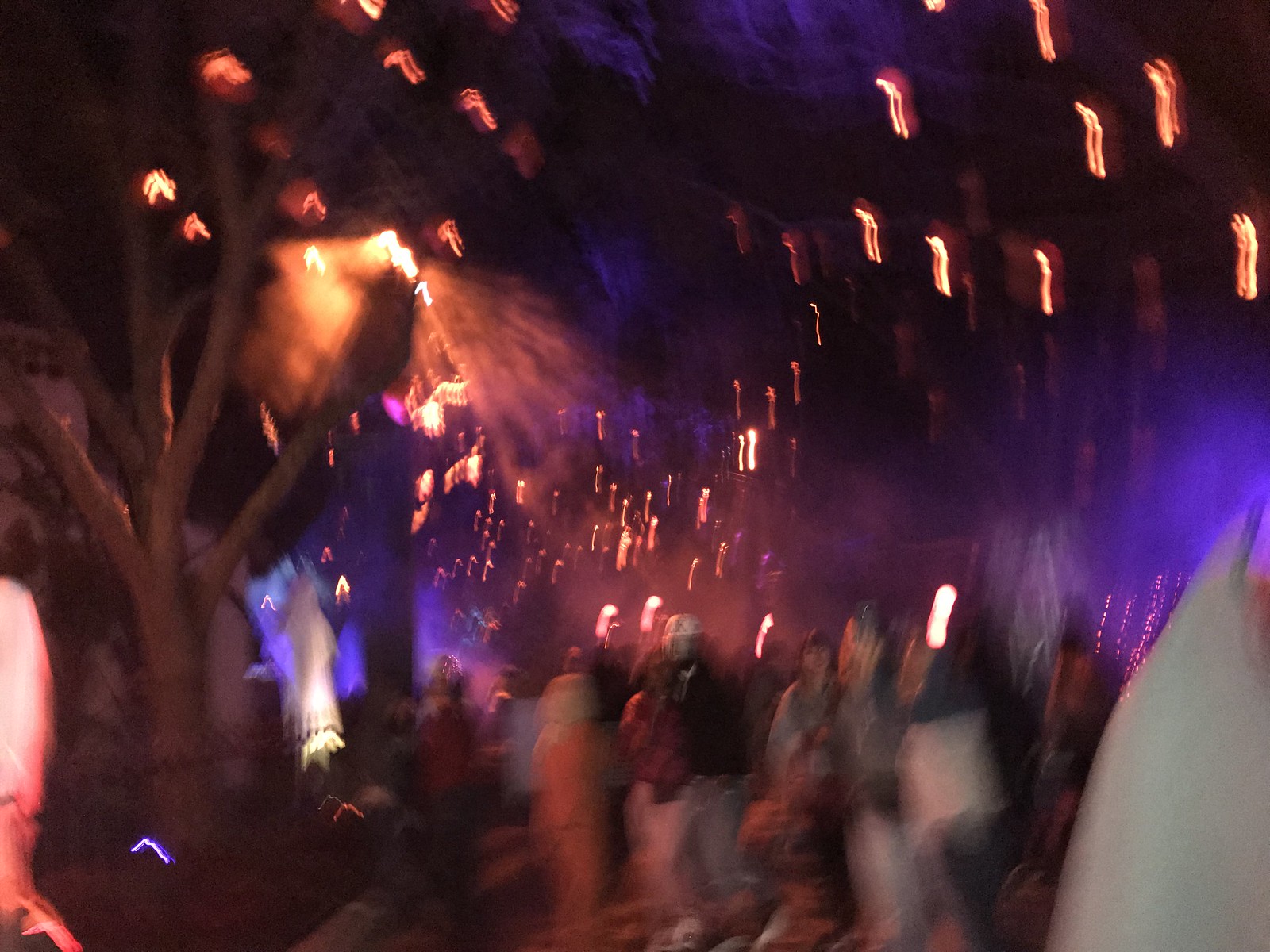The image is a very blurry nighttime scene, possibly from a concert or a party held outdoors. The focal point seems to be a tree with green foliage and brown branches, illuminated by various orange and purple lights. Some of the orange lights appear almost like flames, casting a glowy light at the bottom of the tree and creating squiggly lines throughout the image. There is a pole in the mid-ground and what might be a white sheet hanging from the tree, lending a ghostly appearance, suggesting a possible Halloween theme. Amidst the scene, a crowd of people can be seen, with groups huddled together, some pairs suggesting couples. The overall blur and shaky quality of the photo obscure the details, making it challenging to discern precisely what's happening.